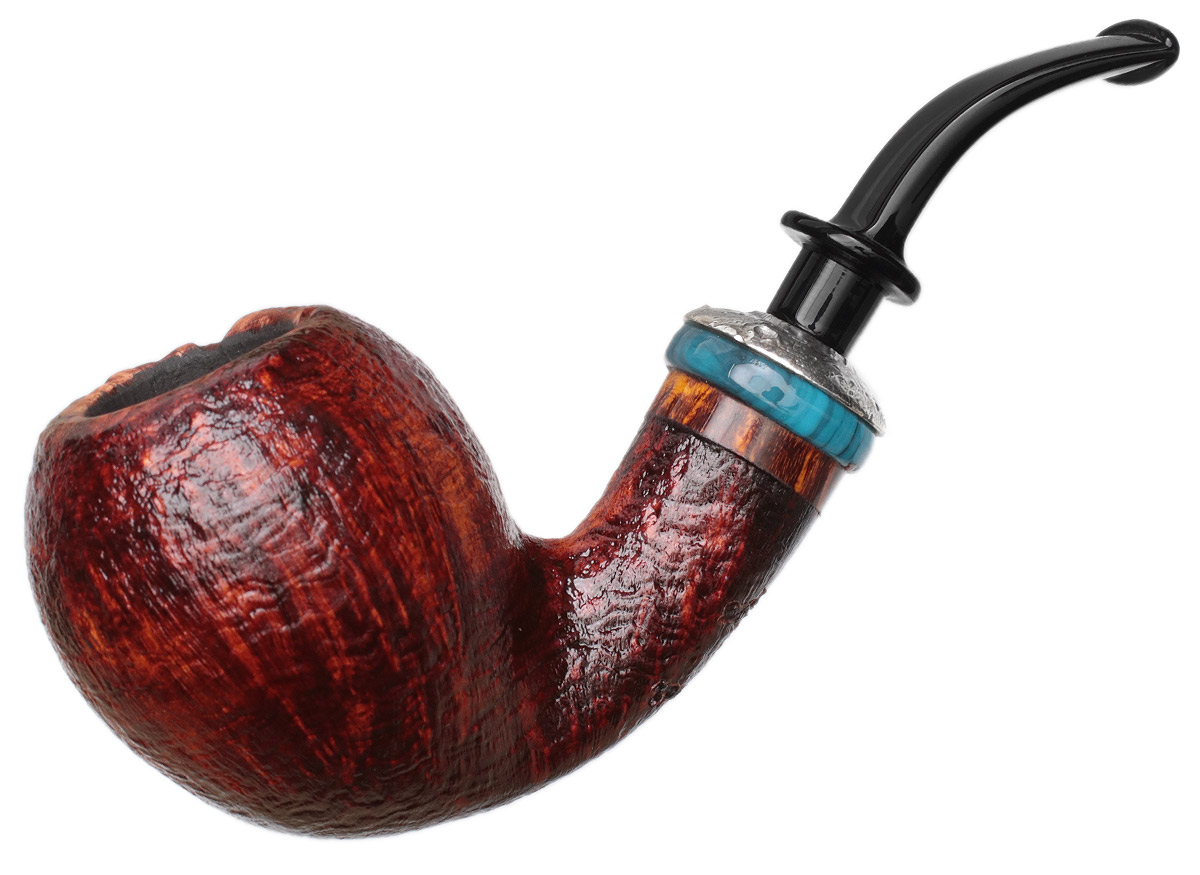This is a close-up color photograph of a vintage tobacco pipe against a plain white background, likely taken in a brightly lit lightbox. The pipe features a shiny black plastic mouthpiece with an oval-shaped end, designed for easy placement in the mouth. This mouthpiece connects to a gleaming silver metal section. Just below this, there's a distinctive donut-shaped, light blue or turquoise band, followed by another band stained gold, blending with the overall wood design. The main body of the pipe is crafted from wood, possibly cherry or walnut, with a rich, deep rust or root beer barrel-like color. The pipe's bowl, or bell, is rounded and curves upward, showcasing a rough texture with streaks of black, indicative of its hand-carved, old-fashioned design. There are no visible text, numbers, or words in the picture, emphasizing the pipe's intricate and vivid color details—brown, black, silver, blue, and gold.